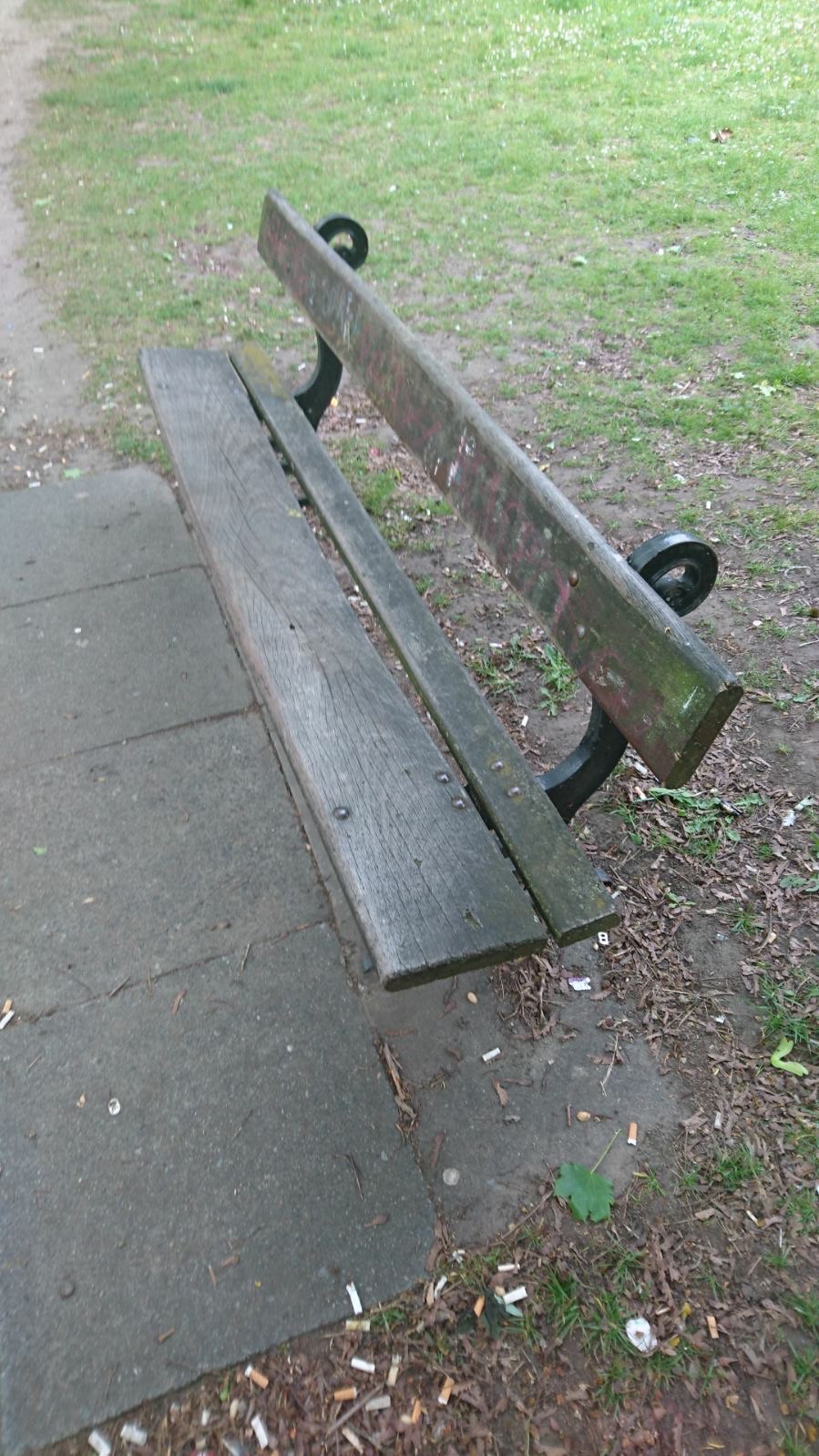The image shows a dilapidated park bench situated on a concrete walkway bordered by patchy, neglected grass. The bench itself is old and poorly maintained, with wooden slats that are warped, stained, and defaced with old graffiti. The single slat backrest and the seat are both dirty, marked with bird droppings, and in need of repainting and cleaning. Surrounding the bench, the ground is littered with cigarette butts and various pieces of trash, contributing to the overall unkempt appearance of the area. The grass around the bench is sparse and mixed with patches of dirt, highlighting the general neglect of the park. The paved walkway leading up to the bench consists of large, evenly cut black stones.